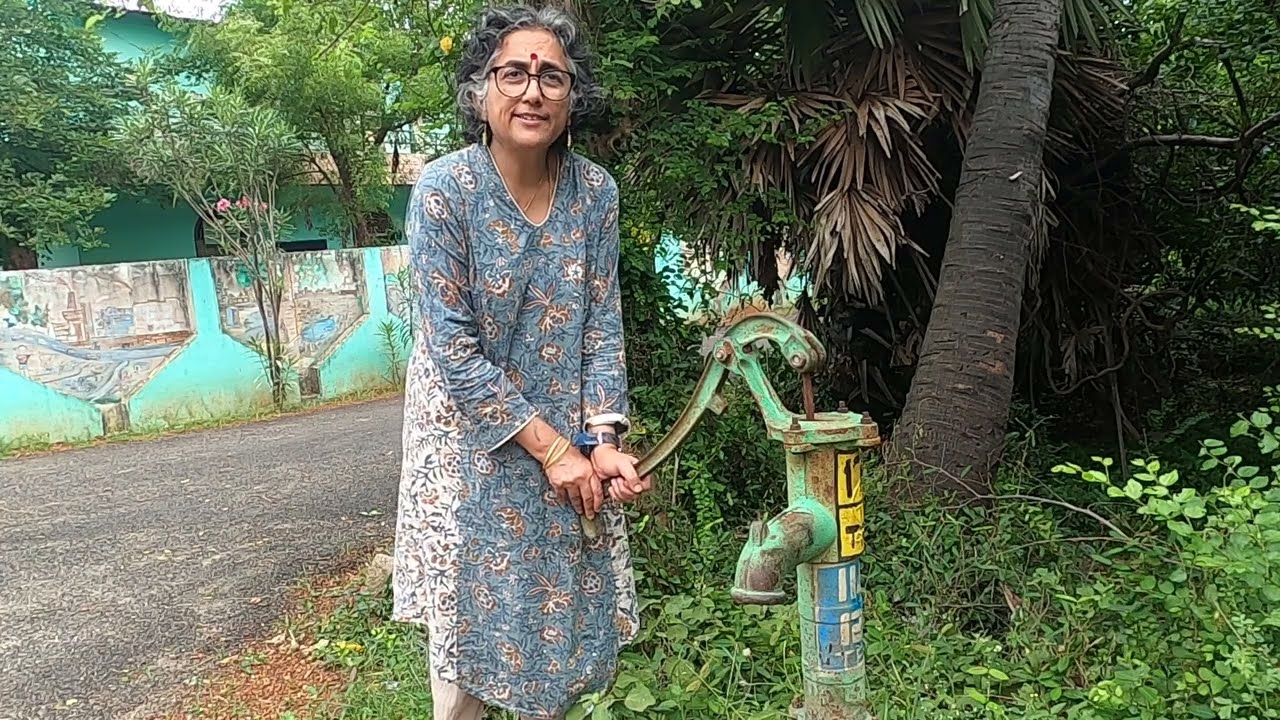This photograph captures an older Indian woman, likely in her 50s or 60s, using a greenish, rusted water pump with stickers on it. She is cranking the handle with her left hand on top and right hand on the bottom. The woman has short, graying hair and wears black glasses. She is adorned with a maroon bindi on her forehead, two bangles on her right hand, and a watch on her left. 

Dressed in a long, dusty blue dress with flower patterns, which appears to be traditional Indian attire, she also wears pants underneath. The scene is set against a backdrop of lush greenery and palm trees, indicative of a tropical environment. To her left is a turquoise green wall with a building painted in a similar bluish-green color behind it. This wall demarcates the edge of a road path.